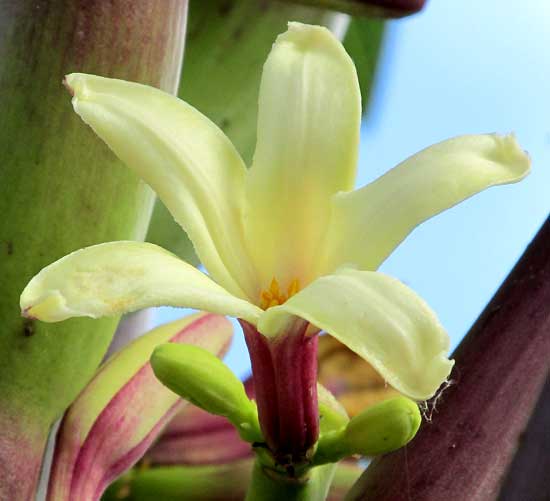This macro color photograph showcases a close-up of a primarily yellowish-white lily. The flower, which is mostly open, displays five prominent petals with a deep bell-shaped bottom. The petals feature a subtle hint of yellow and towards the base, there is a distinctive red hue. Visible within the flower are the reddish stamen and seeds. The green stem of the flower extends from a pink bud, and surrounding the main bloom are several buds and flowers that have not yet bloomed. These unopened flowers are mostly green with slight red tinges on the top and bottom. The background of the image is blurred, featuring more tightly closed lilies to the left, an unidentifiable brownish object tilting to the right, and a faint glimpse of blue sky. The focus is clearly on the intricate details of the lily in the foreground.